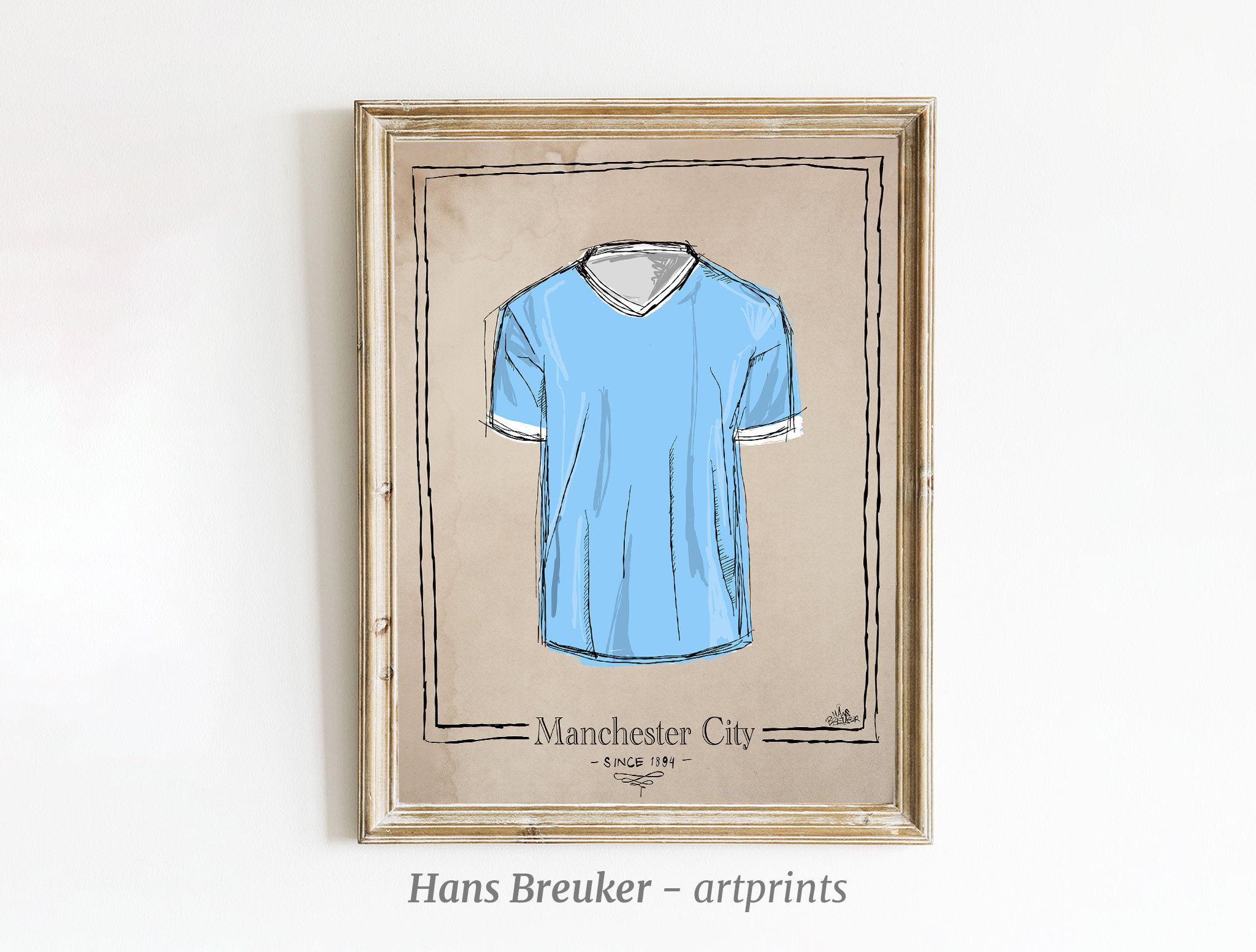This artwork is a framed print featuring an illustration of a blue, short-sleeve, V-neck jersey with white trim around the neck and sleeves, positioned against a beige background. The jersey, which appears to represent Manchester City and its long-standing history dating back to 1894, is surrounded by a subtle, hand-drawn black border. Beneath the illustration, the text in black reads "Manchester City Since 1894," though the exact year is somewhat difficult to discern. Below this, there is another line of text that reads "Hans Bruker Art Prints." The print is set within a distressed tan and white wooden frame and is presented hanging on a white wall. The overall dimensions of the artwork suggest it's taller rather than wide, emphasizing the simplicity and focus on the jersey itself, hinting at a vintage or classic sports memorabilia aesthetic.